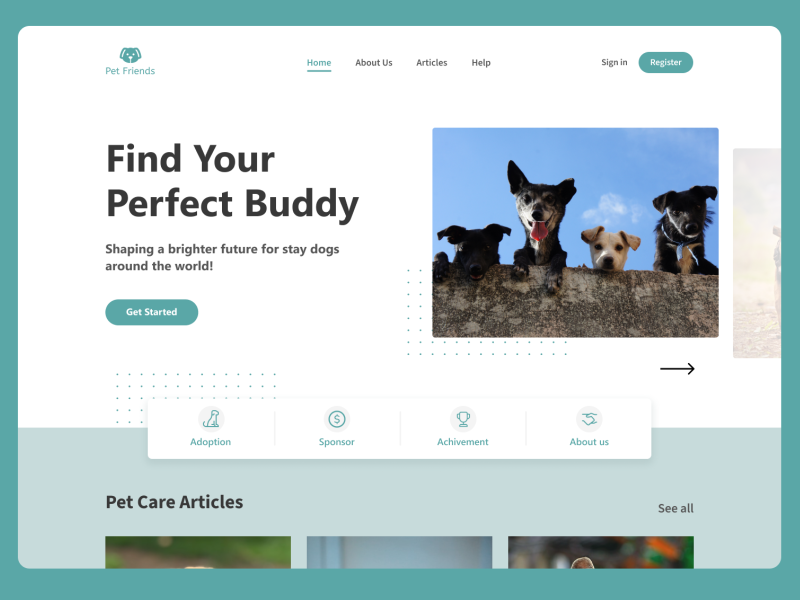This screenshot showcases the homepage of the pet adoption website, Pet Friends. Dominating the top left corner is the site's green logo, featuring a stylized dog head above the text. Central to the header are four primary navigation buttons: Home, About Us, Articles, and Help. The Home button stands out, highlighted in green and underlined, while the others are in black. To the right of this menu are the Sign In and Register buttons, the latter distinguished by its green, pill-shaped design.

Beneath the header, the left side of the screen features bold headline text reading, "Find Your Perfect Buddy," followed by a smaller subhead proclaiming, "Shaping a Brighter Future for Stray Dogs Around the World." Directly below is a prominent green button inviting users to "Get Started."

On the right side, an inviting image displays four dogs peering curiously over a ledge. Below this image, a section presents four icons accompanied by text titles: Adoption, Sponsor, Achievement, and About Us.

The footer includes a friendly message encouraging viewers to contact the site with any questions, stating, "If you have any questions, please feel free to reach out to us. We'd love to hear from you. Thank you."

This detailed arrangement and thoughtful design emphasize the website's commitment to pet adoption and support for stray dogs worldwide.